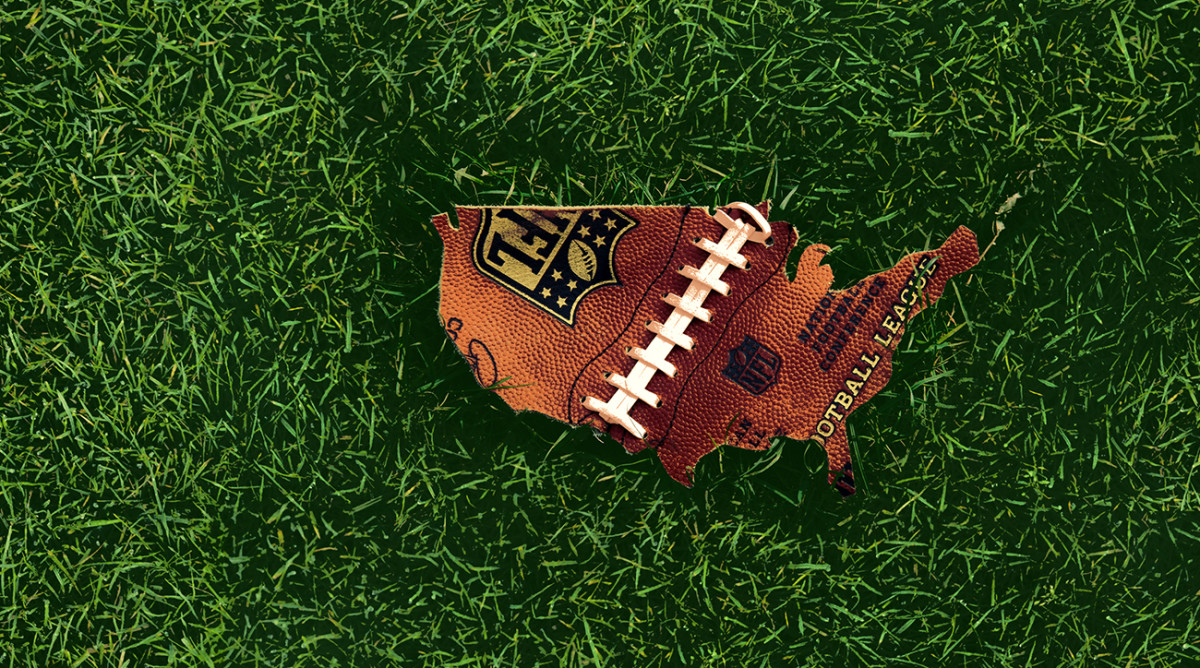In this photograph, a distinctive piece of a football is prominently displayed on a lush, green background that resembles either freshly planted grass or astroturf. The football fragment is meticulously cut, almost resembling the shape of the United States of America. Running down the center of the football are bright white laces that appear to extend from an area mimicking Texas up towards a region around Michigan, with part of the laces seemingly coming undone at the top where the ball was cut. Notably, the leather football bears the emblematic NFL logo and the word "NFL," with a partial gold "Football League" inscription visible. Additionally, there is a section showcasing what looks like part of a signature on the left side of the laces. This unique display combines intricately detailed elements of a classic NFL football with a visually striking, atypical cut, all set against an exceptionally green grassy backdrop.